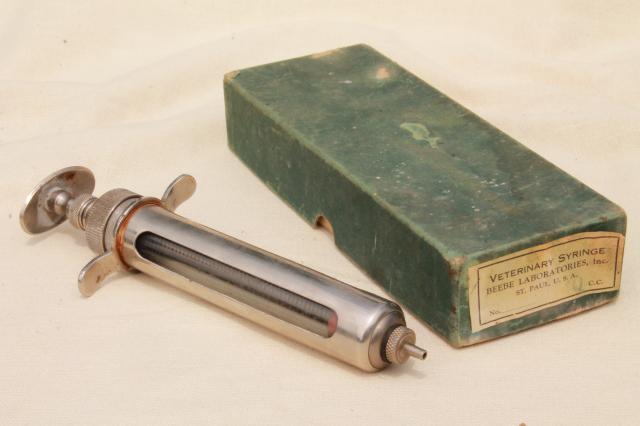The photograph features an antique veterinary syringe and its original packaging, displayed on a white cloth. The syringe, likely from the industrial era of the 1920s or 1930s, is made entirely of metal and exhibits a vintage, industrial design. It has a silver finish and includes two winglet prongs on the sides for finger placement. The syringe is equipped with a glass window to indicate the liquid level inside and a compressed plunger. A hint of red brass coloring can be seen where the finger joints meet the syringe, and slight rust is visible on the plunger.

Adjacent to the syringe is a weathered green box, showing signs of age with scuffed edges, faded color, and a rugged, torn appearance. The box, stamped with a patina, bears a white label bordered in black, reading "Veterinary Syringe, Beed Laboratories Inc., Saint Paul, USA." The label also features a number field and the letters "CC." Despite the wear on the box, the syringe itself remains in relatively good condition, creating a stark contrast between the preserved medical instrument and its aged packaging.